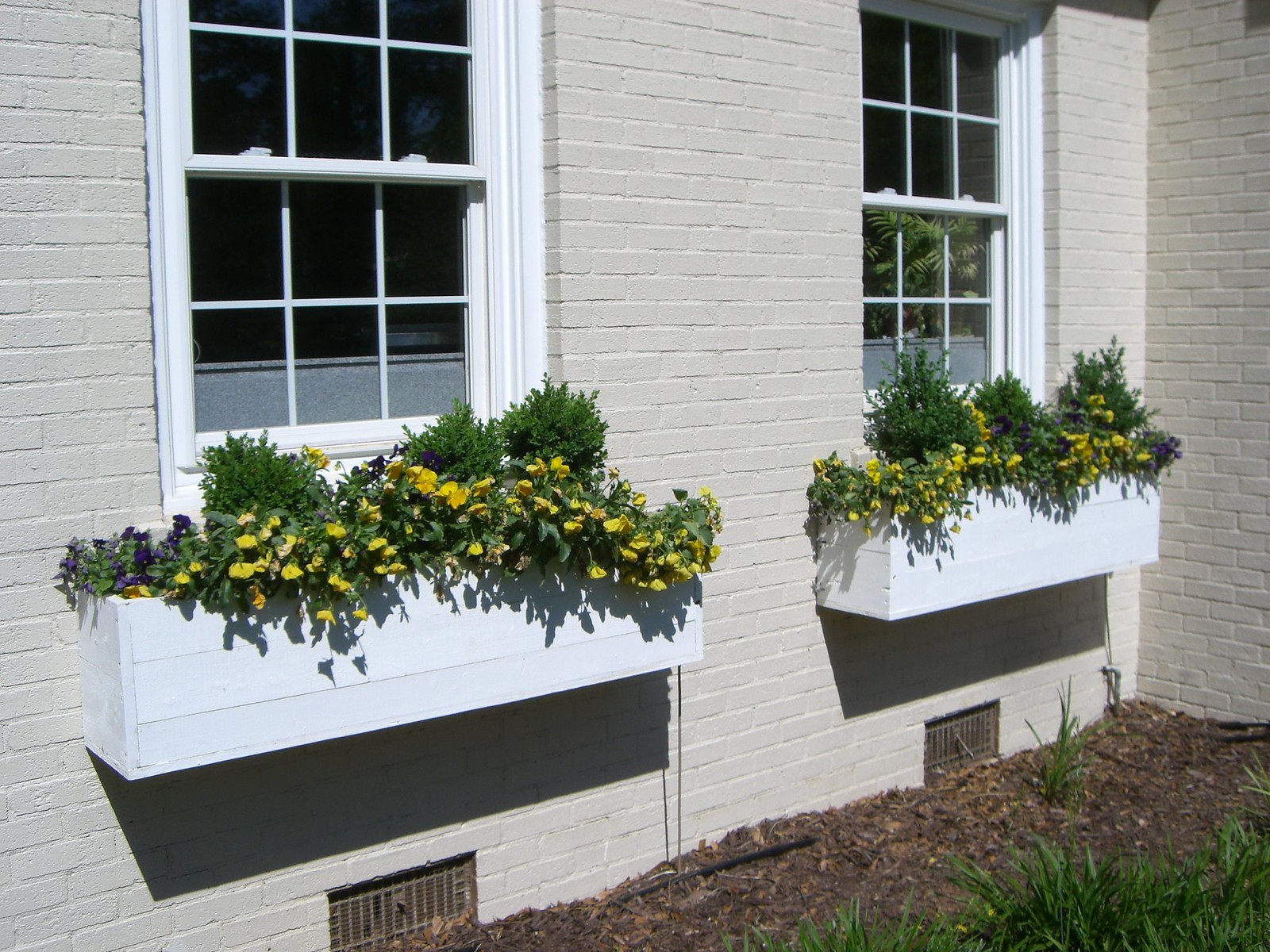This color photograph captures a section of the exterior of a white brick house, highlighting its charming, cohesive design. Two white-trimmed windows with multiple panes dominate the side of the house, each adorned with pristine white wooden flower boxes. The flower boxes brim with vibrant yellow flowers, interspersed with lush green leaves and a few purple blossoms at the edges. The bright daylight casts distinct shadows of the window boxes on the white bricks behind them. Below the windows, a gray border is visible—perhaps the back of a piece of furniture. Beneath this, dark brown mulch lines the ground, where a single clump of grass stands out amidst the mulch. In the lower right corner of the image, the edge of a green lawn is evident. The rightmost window offers a faint glimpse of a plant inside and a reflection of the exterior flora, adding subtle depth to the scene.